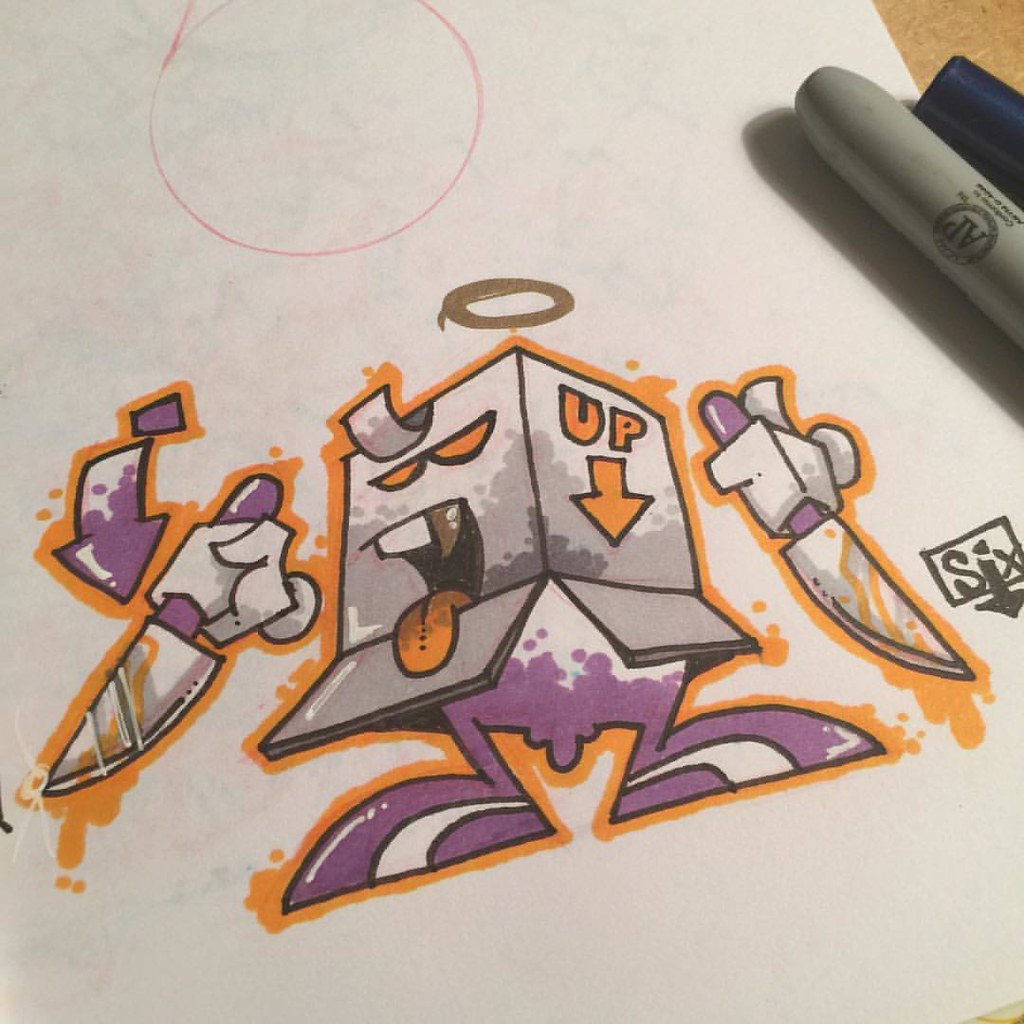The image depicts a whimsical cartoon character set against a white background. At the top right corner of the image, a red circle, possibly made with a marker, contains the letters "AP." The character appears to be constructed from a combination of materials, including cardboard and tape, resembling a handmade or collage-style figure.

The character has a cartoonish face, with distinct orange eyes framed by glasses, and an exaggerated open mouth that reveals one white tooth and one black fang. A tongue sticks out from the mouth, colored in orange. Hovering above the character's head is a halo, adding a humorous or ironic touch.

The character's body is predominantly white and purple. It holds a purple-handled blade in its left hand, which appears to be dripping. An arrow points downwards from the left side of the image, indicating motion or emphasis. The right hand holds another knife, surrounded by orange accents.

An orange border frames the entire image, providing contrast and focus. To the right of the character, there is additional text and a square symbol pointing down with the numeral "6".

Overall, the image gives off a playful and chaotic vibe, blending elements of art and cartoonish exaggeration.